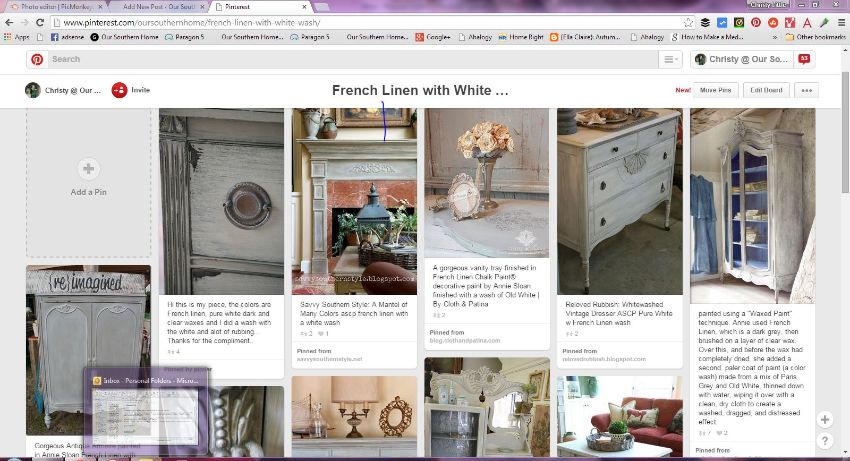This screenshot captures a web page from Pinterest, specifically at the URL "www.pinterest.com/oursouthernhome/French-linen-with-white-wash." The page displays several images showcasing various pieces of furniture finished with a French linen and whitewash technique.

1. **Whitewashed Cabinet**: The cabinet is shown with the heading "re-imagined" written above it, indicating a transformative touch.
2. **Whitewashed Dresser**: Accompanied by a comment that reads, "Hi, this is my piece. The colors are French linen, pure white, dark and clear waxes, and I did a wash with the white and a lot of rubbing. Thanks for the compliment."
3. **Fireplace Setup**: There is an elegant fireplace with a white mantle and a pink granite or marble component above the opening. In front of the fireplace is a coffee table adorned with various knick-knacks, while the mantle holds vases and a painting mounted above it. The caption reads, "Savvy Southern Style: A Mantle of Many Colors," though one word is illegible.
4. **Vanity Tray**: Showcasing a stunning vanity tray finished in French linen chalk paint by Annie Sloan, completed with a wash of old white using cloth and patina. The tray holds a vase and a small framed mirror.
5. **Vintage Dresser**: Described as "Reloved Rubbish," this dresser features a whitewashed vintage aesthetic with ASCP (Annie Sloan Chalk Paint) in pure white, enhanced with a French linen wash. It includes two small drawers on the top and two larger ones on the bottom.
6. **Armoire**: This piece is characterized by its clear glass doors opened to reveal blue-painted shelves within. Created using a wax paint technique, Annie Sloan first applied French linen (a dark gray) followed by a layer of clear wax. Before the wax dried completely, she added a paler color, a mix of Paris gray and old white thinned with water, achieving a washed, dragged, and distressed effect with a clean dry cloth.

Each image embodies the artistic use of French linen and whitewash techniques to enhance and revitalize vintage furniture, reflecting the charm of Southern home decor.